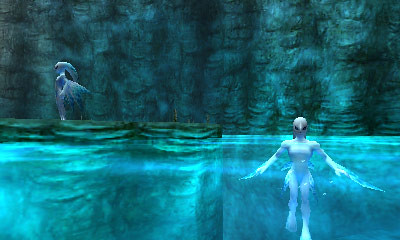The image appears to be a screenshot from a video game, characterized by a predominantly blue and green color palette with dark shades and a teal-like glow. The lower third of the image is filled with translucent, shimmering water that offers a glimpse of the rocks underneath. On the left-hand side, a cliff emerges from the water, rendered in grey, dark green, and dark blue hues. Atop this cliff stands a half-horse, half-bird creature with a striking white and blue body, accented by a long, teal-like structure on its head.

In the lower right-hand corner, a humanoid bird-like creature, with pure white skin, long feathery arms, and a long beak, is treading water. Only the head and shoulders of this female alien-like figure are visible above the surface, with long fins on her arms and sides, and large webbed feet beneath the water. The background of the image features the textured cave walls, contributing to the deep, immersive atmosphere of this otherworldly scene.